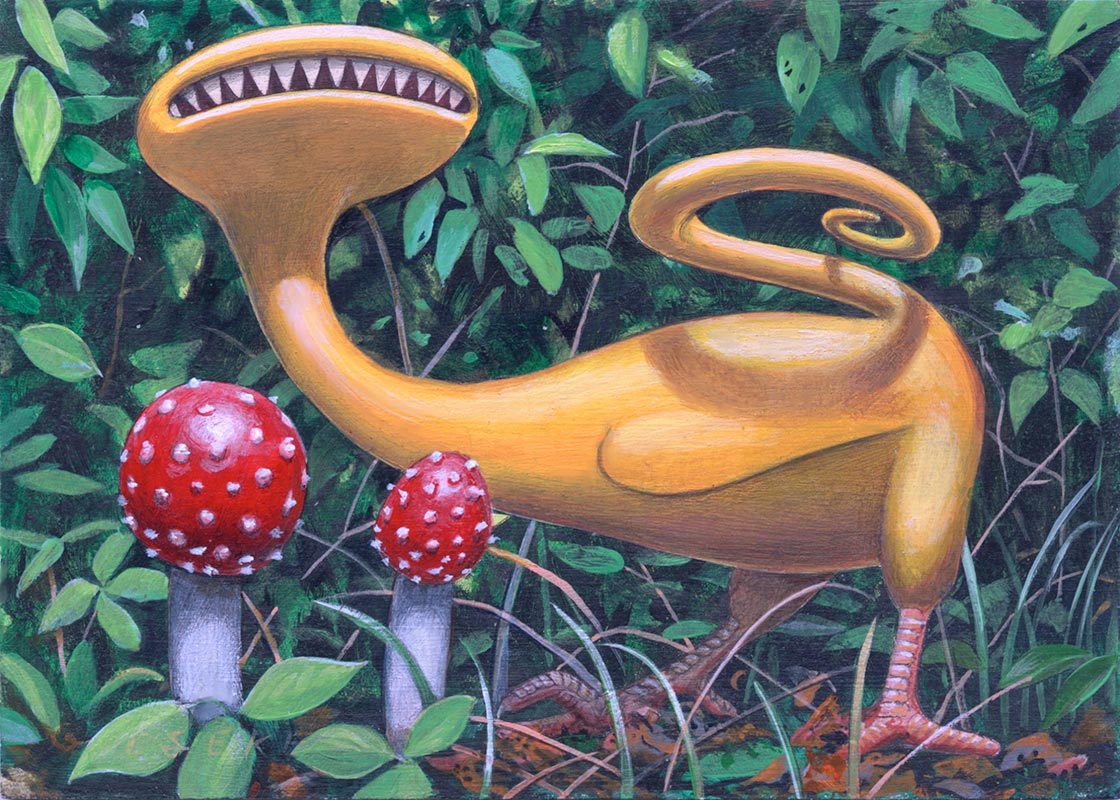The painting depicts a fantastical scene set amidst lush greenery, featuring an animated, predominantly yellow creature as the central focus. This creature has a peculiar, twisted form, reminiscent of multiple animal traits fused together. It stands on bird-like feet with three claws, much like a chicken's, anchored firmly in the ground where longer grass grows. Its elongated, curved neck extends up to a horizontally oval head, notable for its large mouth filled with sharp, white teeth, but devoid of visible eyes, giving it a monstrous appearance.

The creature's orange, curly tail adds a whimsical twist to its form. The backdrop is rich with green foliage, including tall stalks with green leaves and vibrant shrubs, creating a vivid, outdoor setting. In the lower left portion of the image, two distinctive Amanita mushrooms with gray stalks and red caps adorned with small white specks add a touch of whimsy and detail to the scene. The entire composition combines to create a surreal and vibrant illustration, blending elements of fantasy and nature.